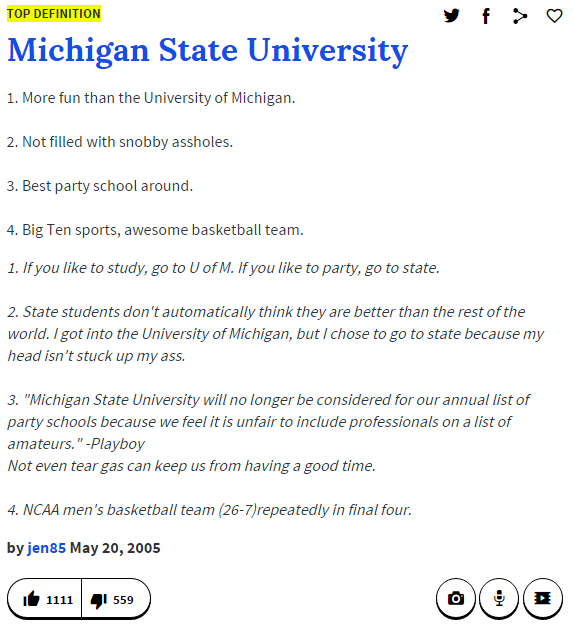The website features "Michigan State University" prominently displayed in large, bold blue lettering at the top. Right above this, "Top Definition" is highlighted in yellow. There are social media icons for Twitter, Facebook, a heart icon, and another icon resembling two lines connecting with circles at their ends.

The content is organized into multiple points:

1. "More fun than the University of Michigan."
2. "Not filled with snobby assholes."
3. "Best party school around."
4. "Big Ten sports and an awesome basketball team."

A grey text annotation below reads, "If you like to study, go to the University of Michigan. If you like to party, go to State." It continues with, "State students don't automatically think they are better than the rest of the world. I got into the University of Michigan but chose to go to State because my head isn't stuck up my ass." 

Another section humorously notes, "Michigan State University will no longer be considered for our annual list of party schools because we feel it is unfair to include professionals on a list of amateurs", credited to Playboy, followed by the statement, "Not even tear gas can keep us from having a good time."

The final point mentions, "NCAA men's basketball team, repeatedly in the Final Four with a record of 26-7." The entire entry is attributed to Jen85, dated May 20th, 2005.